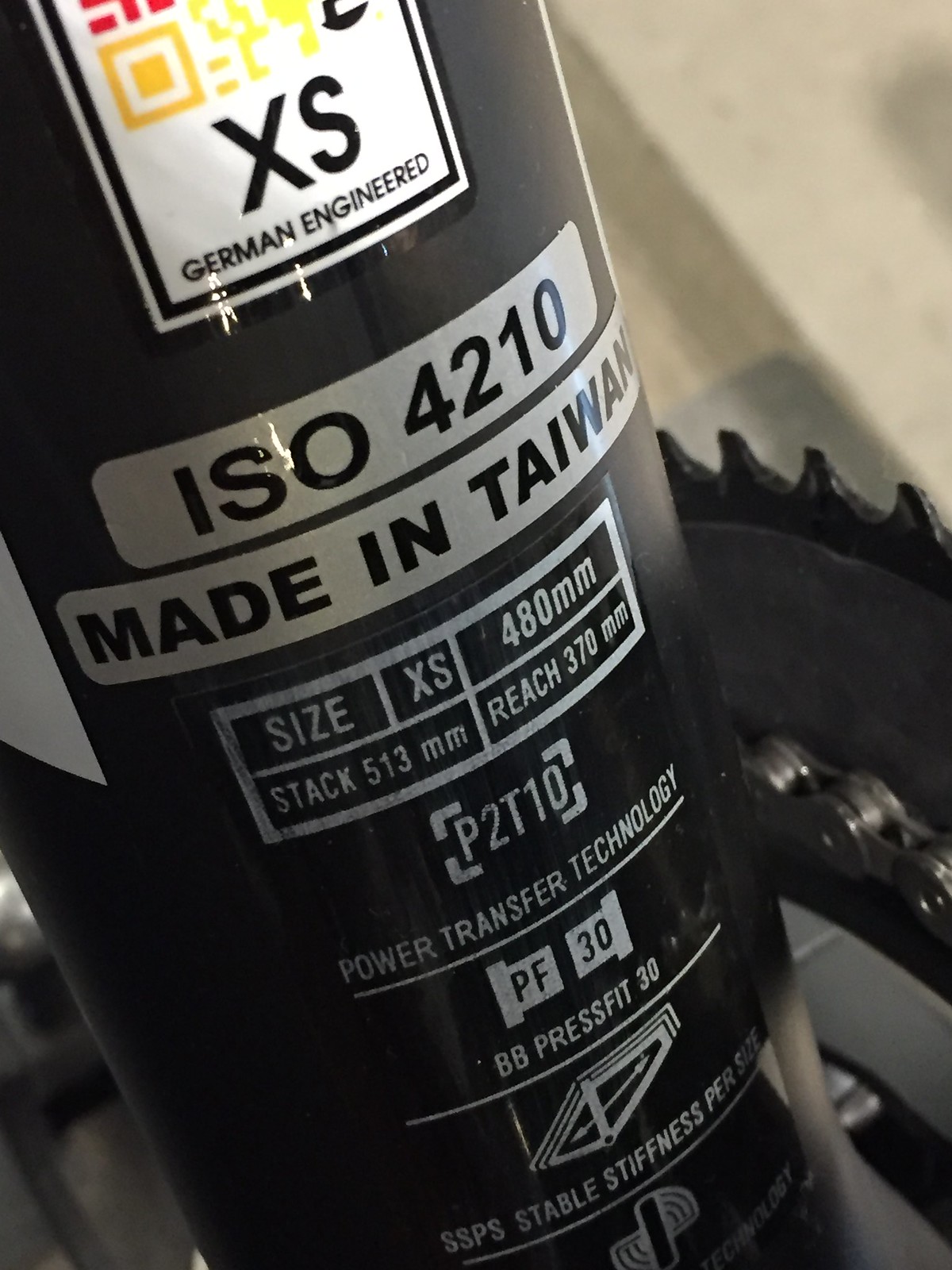The image features a close-up of a black cylindrical canister, potentially a component of an electric bike, embedded within a mechanical setup. This canister has a prominent white label at the top with bold yellow lettering and black text that reads "XS German engineered." Below this, the label specifies "ISO 4210, made in Taiwan," and provides detailed measurements: "size XS 480mm, stack 513mm, reach 370mm." It also touts "P2T10, power transfer technology, PF30, BB, press fit 30, SSPS, stable stiffness." To the right of the canister, there are metal links and a black blade resembling a saw, indicating a connection to mechanical or power transfer functions. The background includes a black piece of metal to the left of the canister and a white surface with dark patches, located in the upper-right corner, possibly part of a wall or roof. The surrounding elements, including visible gears and chains, suggest that this canister is an integral part of an electric bike's drivetrain or motor system.